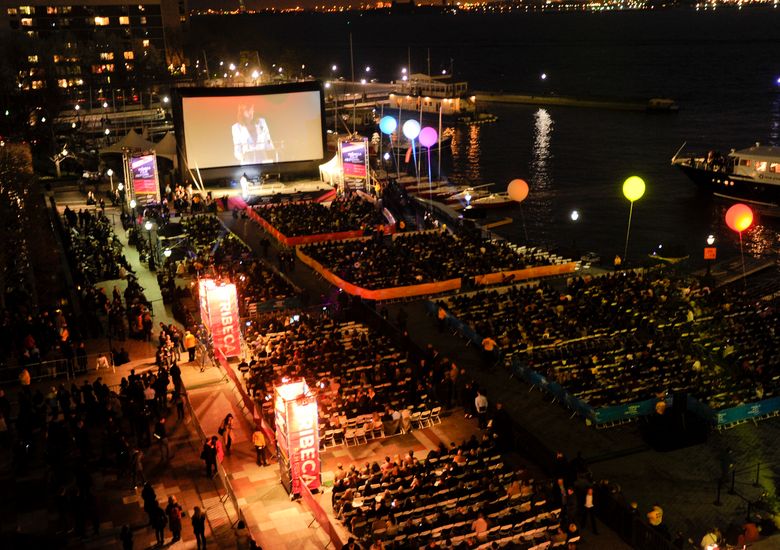The image depicts a nighttime scene at the Tribeca Film Festival, set along the edge of a waterway. The centerpiece of the image is a large movie screen displaying a woman dressed in a white suit, who is also seen live on stage in front of the audience. This outdoor event features several rows of seated attendees watching and listening attentively. Large, colorful balloons resembling neon lights hover above the crowd, adding a festive atmosphere. In the background, you can see yachts and ferries on the water, along with lighted buildings and a pier extending into the water. Tall, illuminated signs in red and white bearing the name “Tribeca” are positioned between the seating areas, emphasizing the event's branding. The surrounding urban landscape and artificial lights illuminate the scene, highlighting the boardwalk and creating a vibrant night-time ambiance.